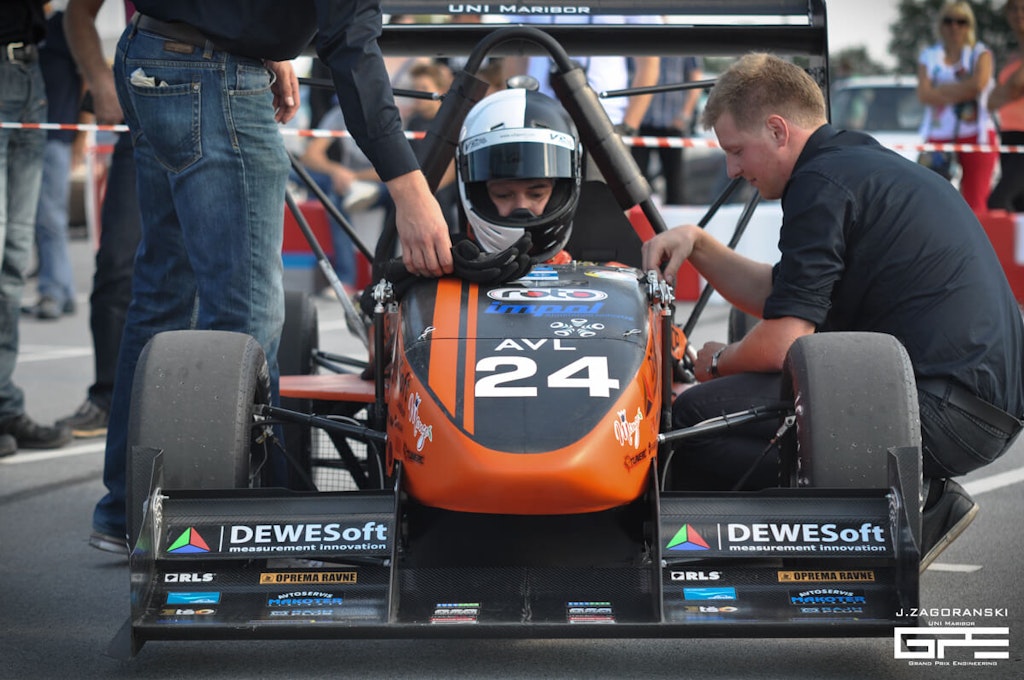The photograph depicts an outdoor scene at a race track, featuring a sleek, orange race car with number 24 prominently displayed on its hood. The car resembles an elevated go-kart with a tubular, narrow body and smooth tires. Its black bumper and rear spoiler, along with the text "DUSOFT Measurement Innovation" signify sponsorship. The driver, seated in the car, is outfitted in a full protective suit and a striking black and white helmet with a black visor, which is raised. He appears to be a young individual or small child, focused downwards.

Flanking the car are two men, engrossed in preparatory activities. One man, crouched to the car's right, has short brown hair and is wearing blue jeans with a dark shirt. Another man, partially visible to the left, sports jeans, a black long-sleeve shirt, and has placed his gloves on the car's hood. Behind them, a blurred crowd stands behind a rope barrier, observing the scene on what appears to be a bright and pleasant day. The watermark "JZagoranski" subtly marks the photo's lower side, alongside a faint label that might read "GPS" in an unusual font.